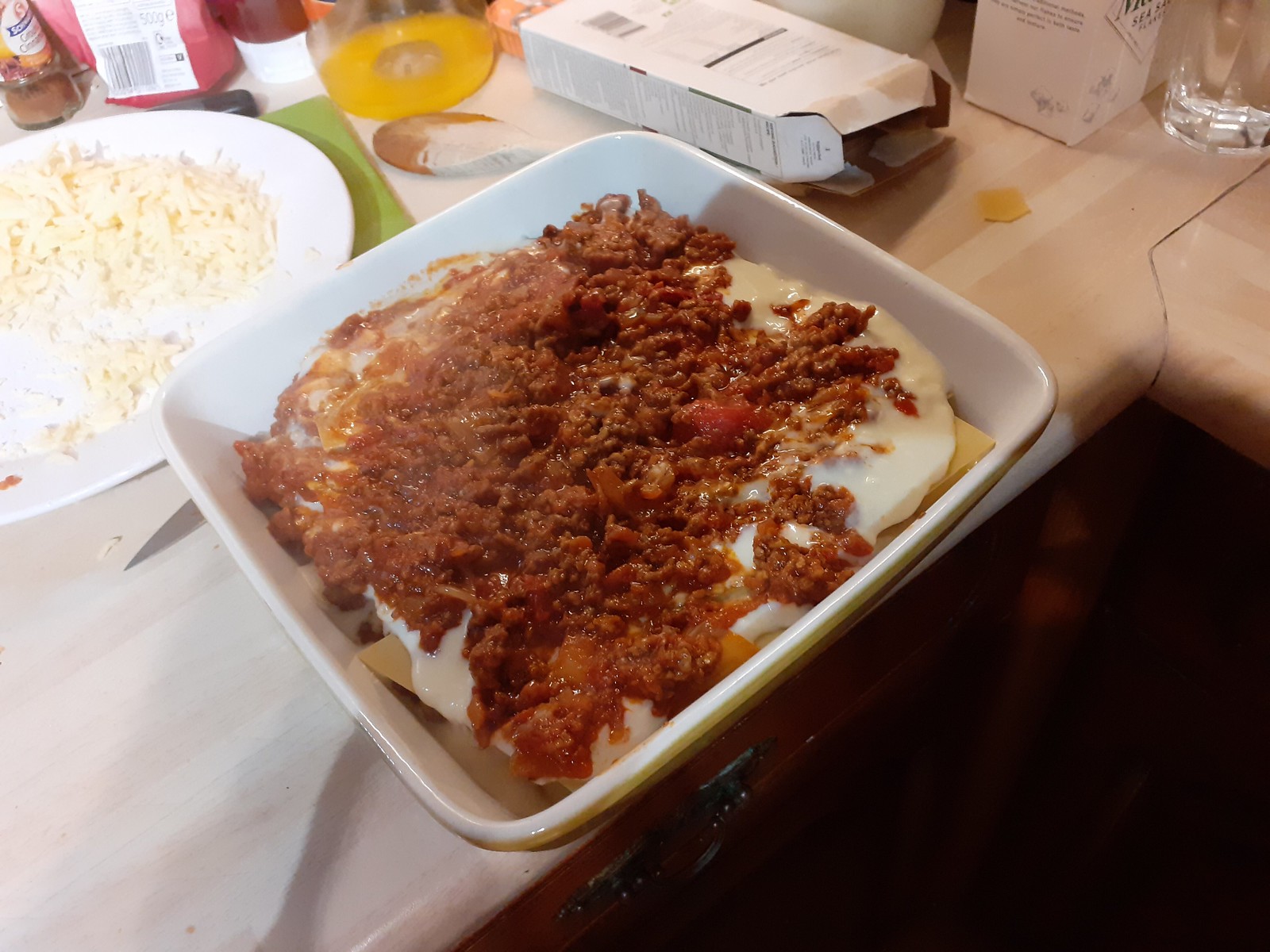In this detailed image, we observe a bustling kitchen scene with evident meal preparation. The countertop is a light-colored, tan wood with an off-white striping, extending to a corner where it meets a darker reddish-brown cabinet. Dominating the center of the image is a square, white ceramic dish brimming with lasagna - featuring layers of wide pasta noodles, ground beef, red tomato sauce, and melted yellow cheese. Adjacent to this, on the left, lies a round plate of white rice.

A white bowl at the image's edge contains a brown mixture with flecks of white and a topping of yellow cheese. Scattered around are various kitchen items: a clear glass filled with yellow juice, a wooden spoon with a white-tipped end, a paper bag labeled "500g" in black text on a red background, and a bottle with a brown substance and a white label. In the right corner, there's a white cardboard box lying open above brown shelves adorned with black metal handles. The background of the scene also includes some additional boxes and items that contribute to a somewhat cluttered but lively preparation area.